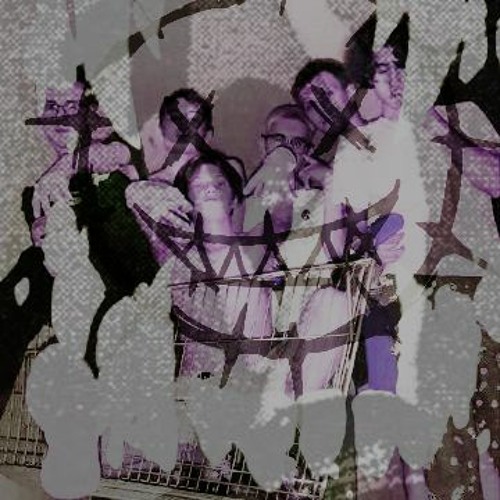In this mixed media artwork, a black and white photograph of six males, tinted with a deep purple hue, serves as the base. The group appears to be posing with a shopping cart, engaged in playful gestures. One man on the left is identifiable by his black shirt and glasses, while another individual on the right wears a white t-shirt and has floppy brown hair. Overlaid on this photograph is a graphic design of a sinister, grinning face with fangs and X's for eyes, which strategically covers the faces of two of the men in the photo. The background is textured with white paint splatters and black spots, adding to the chaotic visual effect. This combination of detailed elements contributes to an overall surreal, almost devilish, aesthetic.